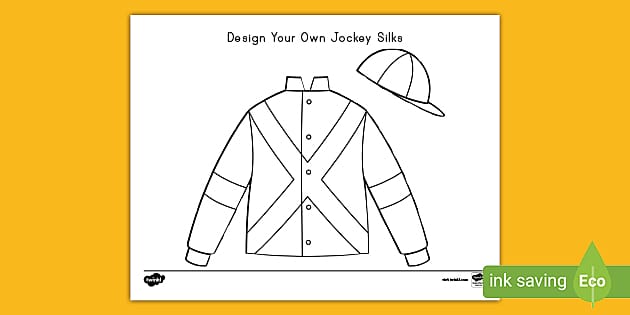The image is a black-and-white drawing on a white piece of paper, showcased against a yellow background. At the top of the paper, bold black text reads "Design Your Own Jockey Silks." The drawing includes a simple outline of a jockey’s jacket and a baseball cap. The jacket is styled like a bomber jacket, featuring a double line X across the front and a stripe halfway up the long sleeves, which end in cuffs. There are buttons on the right-hand side of the jacket. The baseball cap, positioned to the right of the jacket, has two stripes running down the center and a brim. In the bottom left corner of the image, there is a graphic labeled "Ink Saving Echo," with "echo" inside a green water drop shape.